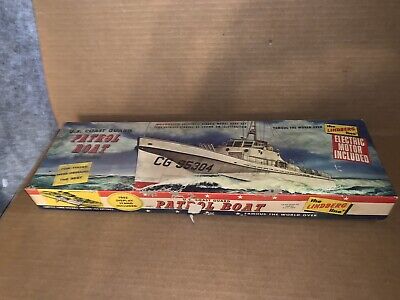In this detailed photograph, a vintage toy box is prominently displayed. The box, which is placed on a corrugated brown cardboard base, appears quite aged and possibly from the 1950s, suggested by its retro color scheme. It features a long, shallow design with striking yellow and red accents. The top of the box is adorned with the text "Patrol Boat" and highlights that an electronic motor is included. There's a starburst emphasizing specific features of the toy, although much of the smaller text is hard to decipher.

The box depicts a dynamic scene where a white patrol boat, marked with "CG 96304" in black lettering, sails through crashing waves beneath a blue sky with scattered clouds. The boat also features a red underside. Additional design elements include red and white decorations, along with smaller yellow labels around the sides. The overall impression is one of vintage nostalgia, with the packaging serving as a lively advertisement for what appears to be a model kit, possibly requiring assembly, by the Lindbergh company. It seems the photograph was taken to showcase the item, possibly for sale, accentuating its collectible and historical value.